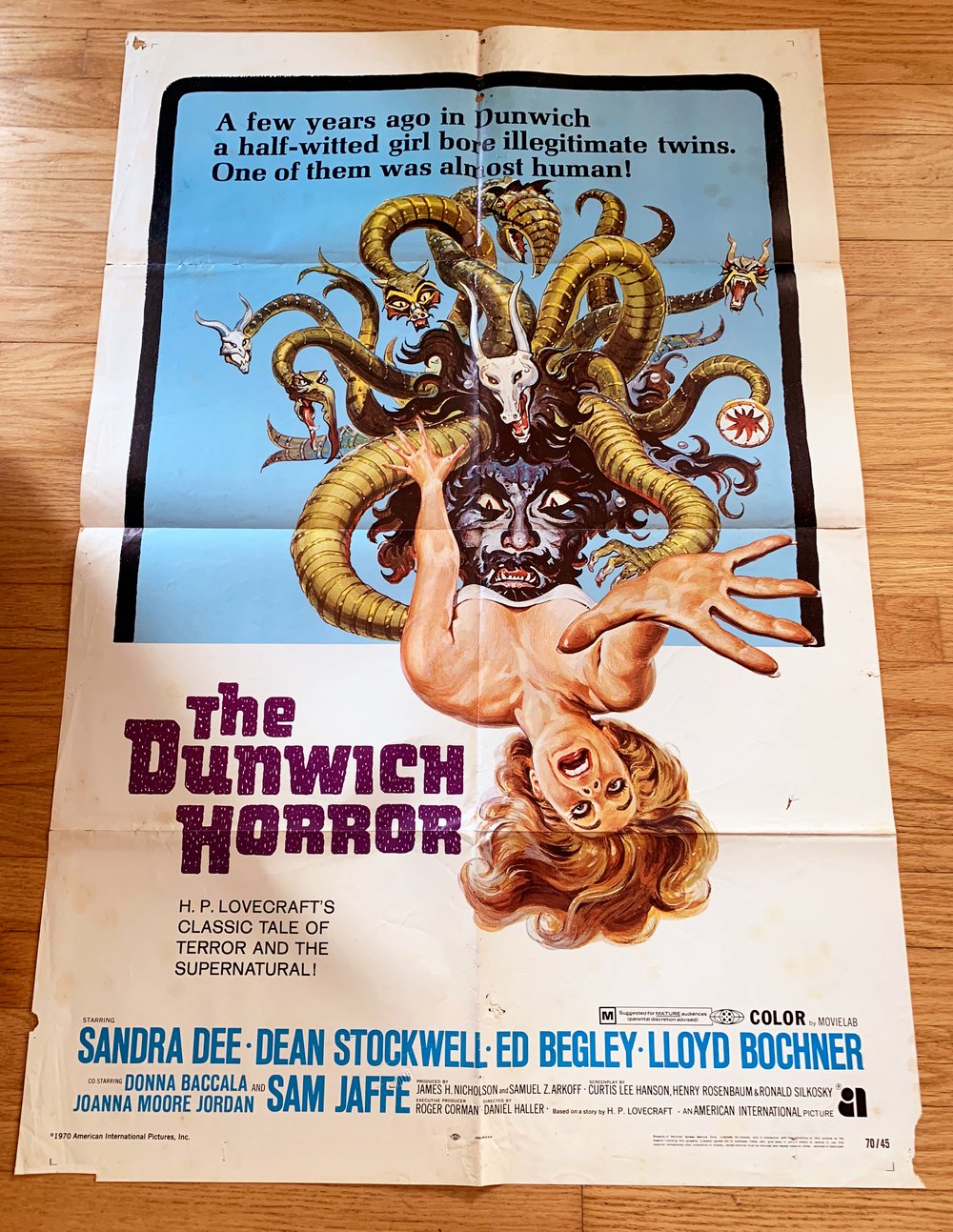This image is a detailed photograph of a vintage movie poster for "The Dunwich Horror," a film likely from the 1960s or 70s, based on H.P. Lovecraft's classic tale of terror and the supernatural. The tall, rectangular poster is laid out on a wooden surface featuring narrow, light brown horizontal panels. The bottom of the poster appears more visible and wider due to the camera angle.

The white paper poster shows signs of aging, including fold lines that divide it into eight squares and slight tearing at the edges, suggesting it was previously folded and perhaps pinned on a wall. The top section of the poster features a bold, blue rectangular portion bordered with a thick black line. This section reads: "A few years ago, in Dunwich, a half-witted girl bore illegitimate twins. One of them was almost human."

Below this text is an illustration of a sinister creature with snakes and horns, resembling a devil with wide, piercing eyes and fangs. The creature's head has tentacles with various creatures at their tips, such as cats, birds, and dragons. This terrifying figure looms over a young blonde woman, who is screaming with her arms outstretched in a desperate attempt to fend off the fiend. Her head and hair appear inverted, adding to the chaotic scene, as one hand pushes back against the creature and the other reaches outwards.

At the very bottom of the poster, the cast is listed, including Sondra Dee, Dean Stockwell, Ed Begley, Lloyd Bochner, and Sam Jaffe, who may be the director. Other credits are too small to discern clearly. The photograph captures the aged beauty of the poster, invoking a nostalgic look at this horror classic.